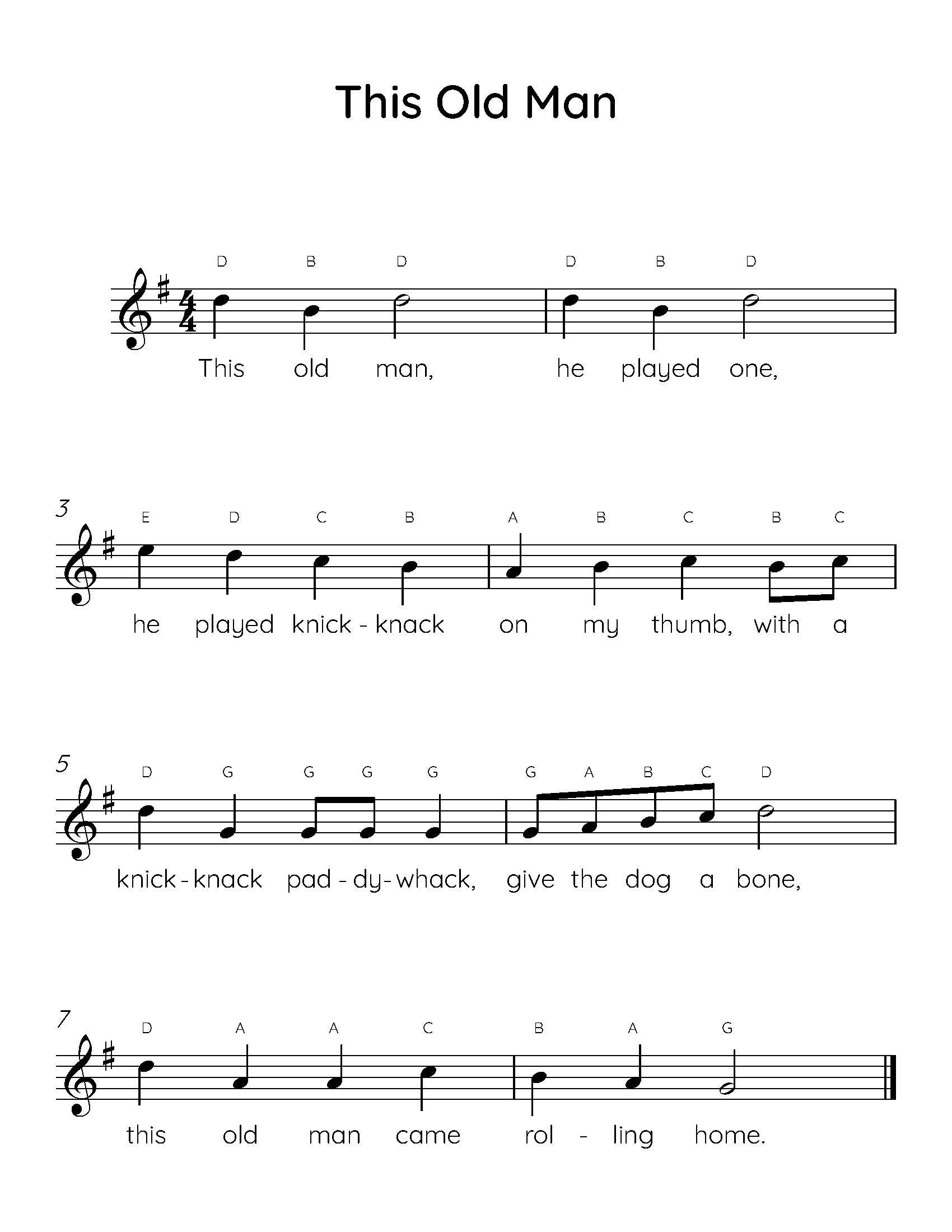The image depicts a sheet of music for the song "This Old Man," displayed on a white background in black and white. The title, "This Old Man," appears prominently at the top in bold text. The music is arranged in four bars, with each bar containing the corresponding musical notes and lines, along with the lyrics positioned beneath them to indicate their alignment with the notes. The lyrics read: "This old man, he played one. He played knick-knack on my thumb. With a knick-knack paddywhack, give the dog a bone. This old man came rolling home." Additionally, some bars feature numbers at the end, specifically three, five, and seven, and each musical note is annotated with its corresponding letter.